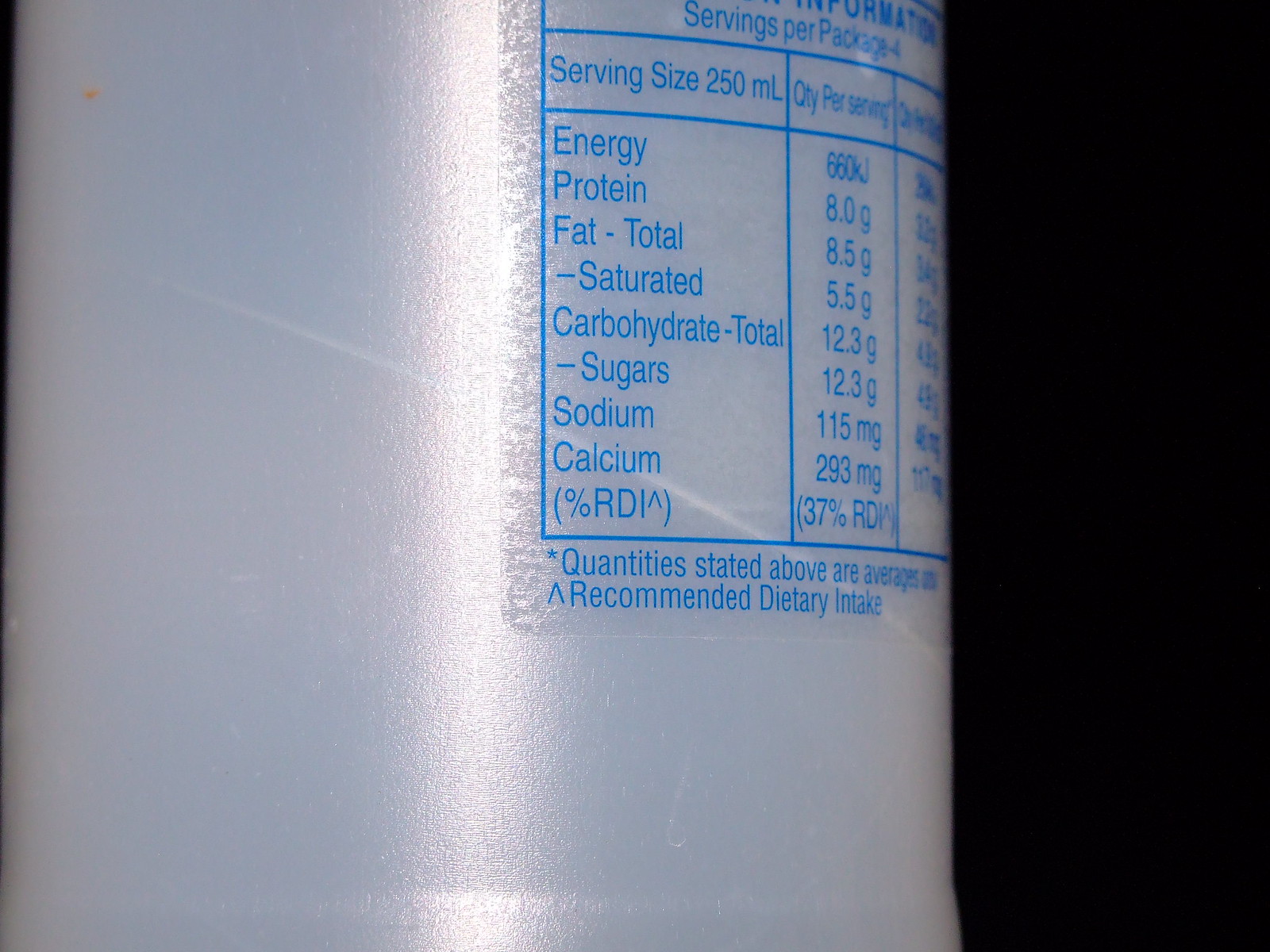The image displays the nutrition label on the back of a frosted, translucent plastic container, possibly a bottle or tube. This indoor color photograph shows the label slightly off-center to the right, against a background where the right third of the image is mostly black. A light glare can be observed just left of center on the container. The nutrition label, which takes up about 80% of the image, is set in a large blue square with several horizontal lines dividing it into smaller sections.

At the top of the label, it mentions "Servings per package: 4" and "Serving size: 250 milliliters." Below this, the label lists various nutritional components in blue text, including "Energy," "Protein," "Fat," "Total Fat," "Saturated Fat," "Carbohydrate," "Total Sugars," "Sodium," and "Calcium," accompanied by their respective values. Additionally, in parentheses next to each component, it indicates "% RDI" (Recommended Dietary Intake) with a caret symbol.

An asterisk at the bottom specifies that the stated quantities are averages. The container itself is frosted plastic, contributing to its translucent appearance.